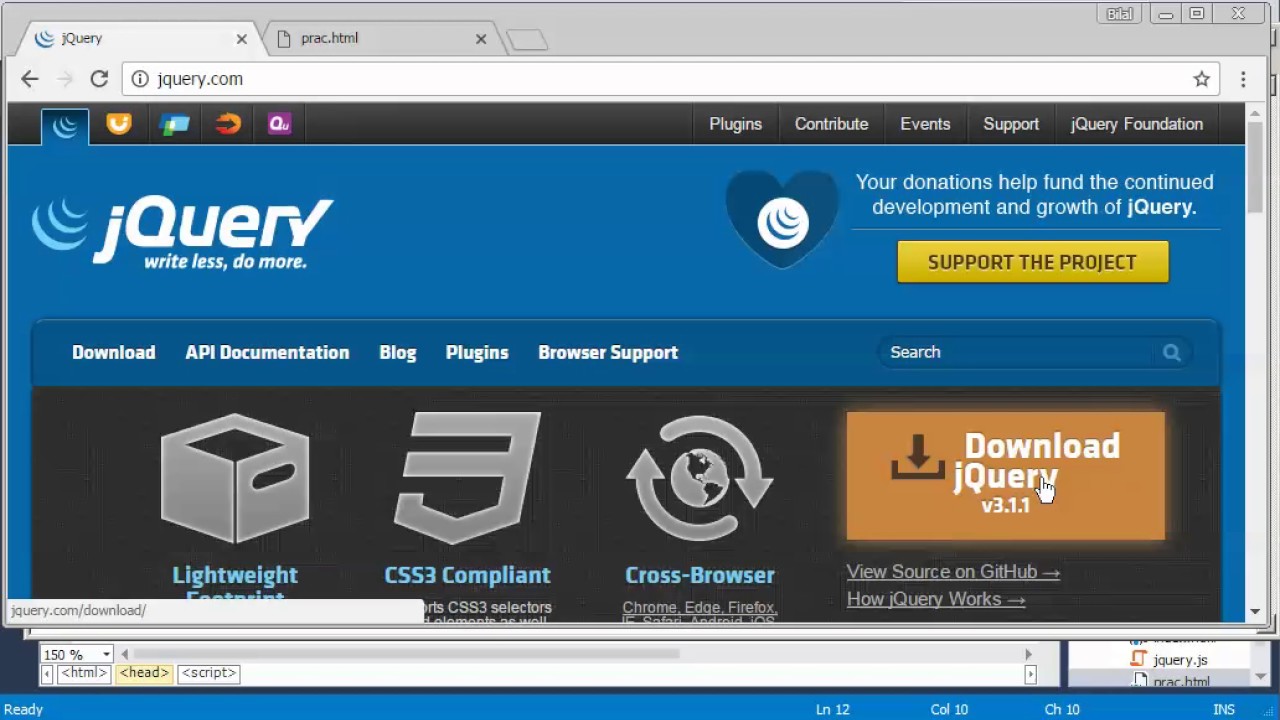The image depicts a web browser screen grab showcasing a website related to jQuery. The image has a landscape orientation, being approximately 50% to twice as wide as it is tall. 

The browser interface displays two tabs at the top: the active tab labeled "jQuery" and a background tab labeled "prac.html." Beneath the tabs, traditional browser navigation buttons are visible, including back, forward, and refresh, followed by the URL bar showing jQuery.com.

The main content of the screenshot presents the jQuery website interface against a medium blue background. At the top of this section, there are several navigation icons and menu options on a gray background with a black foreground. These menu options include "Plugins," "Contribute," "Events," "Support," and "jQuery Foundation."

Towards the upper left-hand side of the main area, the website prominently displays the text "jQuery. Write less, do more." On the upper right-hand side, a dark blue heart icon is visible, adjacent to a message in gray text that reads, "Your donations help fund the continued development and growth of jQuery." Below this message, a yellow button with black text encourages users to "Support the project."

Further down, additional menu options are listed, such as "Download," "API Documentation," "Blog," "Plugins," and "Web Browser Support."

Overall, the image efficiently encapsulates the layout and main elements of the jQuery website within the confines of a typical web browser interface.